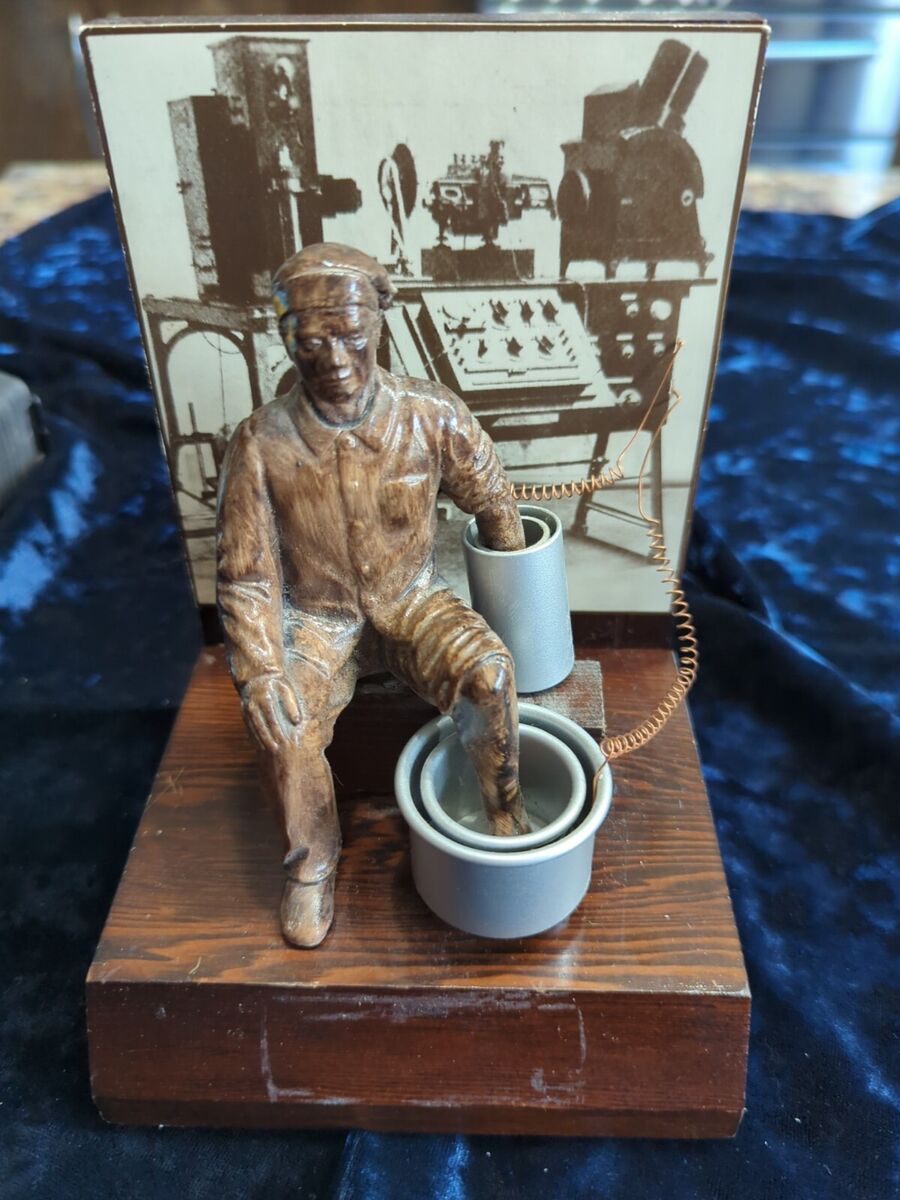This full-color photograph, seemingly taken indoors with a mix of artificial or natural light, depicts a museum-like exhibit set against a textured, crushed blue velvet cloth backdrop, which is draped unevenly creating noticeable folds and wrinkles. Occupying the foreground, there is a detailed wooden sculpture of a man sitting on a medium brown wooden block with visible wood grain. The man wears a hat and has his right pant leg scrunched up past the knee, with his foot inserted into a white ceramic cylinder linked by copper wires to an old black and white photograph behind him. His arm is similarly immersed in another white cylindrical object, also connected by wires to the photograph. The photograph, propped up behind the sculpture, features an indistinct piece of antique machinery on a desk. In the distance to the right, blurred into the background, you can faintly discern a window reflecting light, adding to the scene's ambiance.